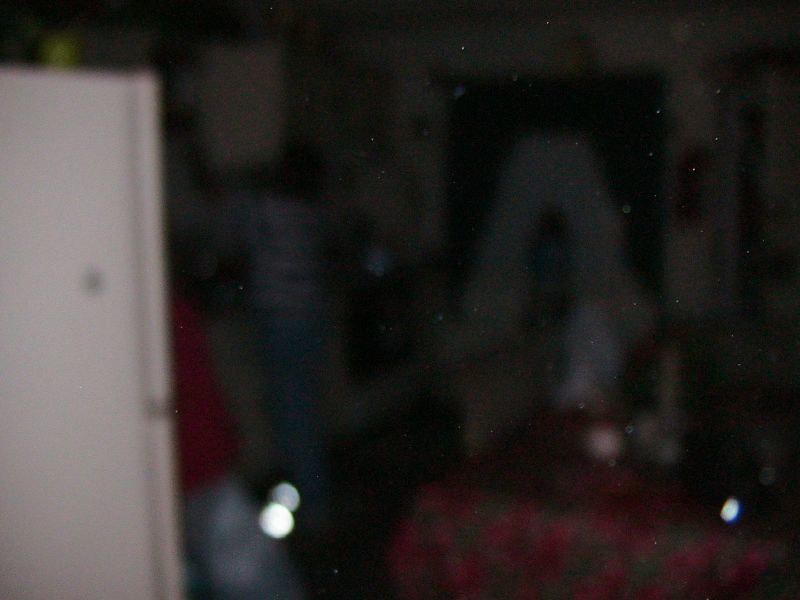In this blurry photograph, the predominant feature is a dimly lit background occupying approximately four-fifths of the image, characterized by dark hues interspersed with grayish streaks and a few small, circular white reflections. These elements contribute to an overall obscure ambiance. On the left side of the image, starting from the lower left corner and extending almost to the top, there is the discernible side profile of a white refrigerator. The design of the appliance indicates it has a top section that is twice as tall as the lower part, implying that the refrigerator compartment is on top and the smaller freezer compartment is at the bottom. This assessment is based on the visible narrow doors, which run vertically from the top to the bottom of the refrigerator.